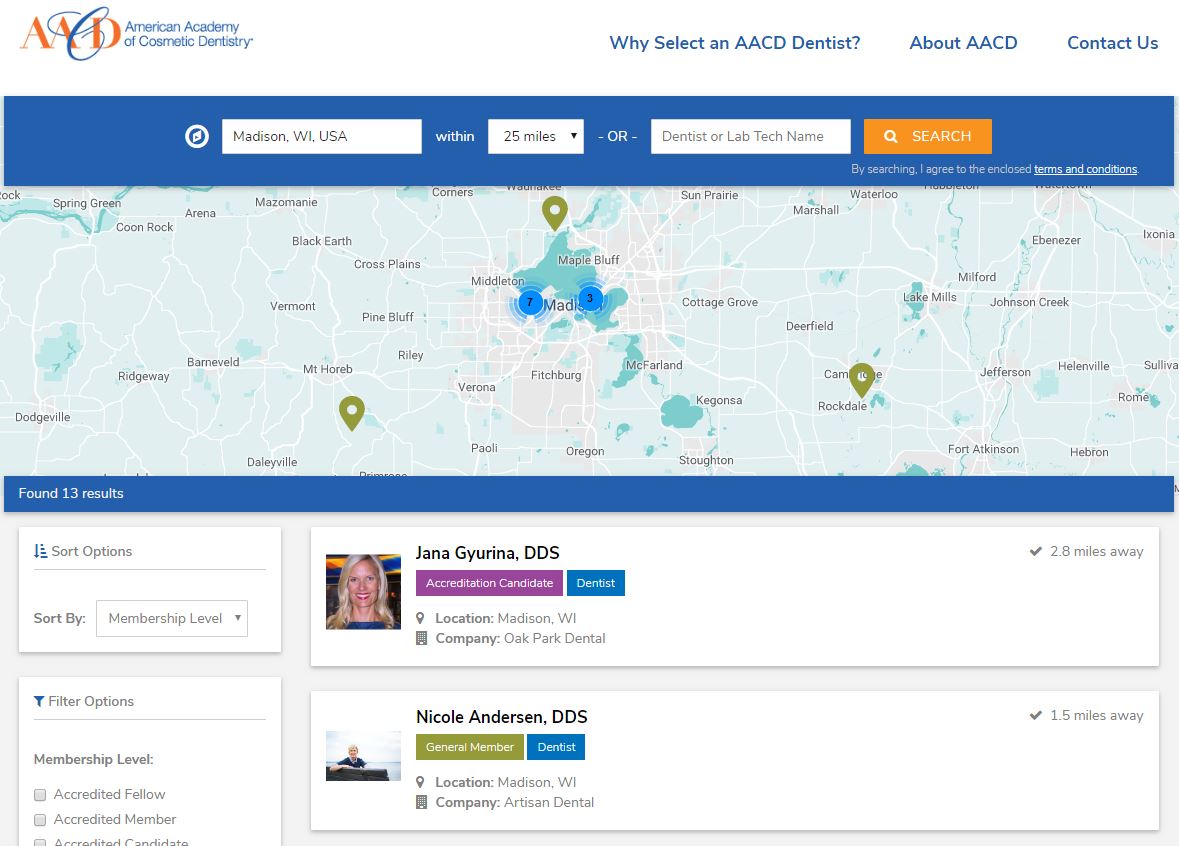The image features a website interface with a primarily white background, prominently displaying the logo and name "AAD American Academy of Cosmetic Dentistry" at the top. Below this header, there is a navigation menu with the options "Why Select an AACD Dentist", "About AACD", and "Contact Us".

Beneath the menu is a dark blue search box. The search function includes text fields where "Madison, Wisconsin, USA" is entered, followed by a drop-down menu set to "25 miles." Additionally, there is a text box labeled "Dentist or Lab Tech Name". An orange "Search" button is located next to these fields. 

The section below the search bar features a map of Madison, Wisconsin, marked with three green location pins. Two blue circles on the map are highlighted with the numbers "7" and "3" inside them. 

At the bottom of the map, the text indicates that "13 results" were found, with one specific result detailed as "Jaina Giurina, DDS - Accreditation Candidate, Dentist," located in Madison.